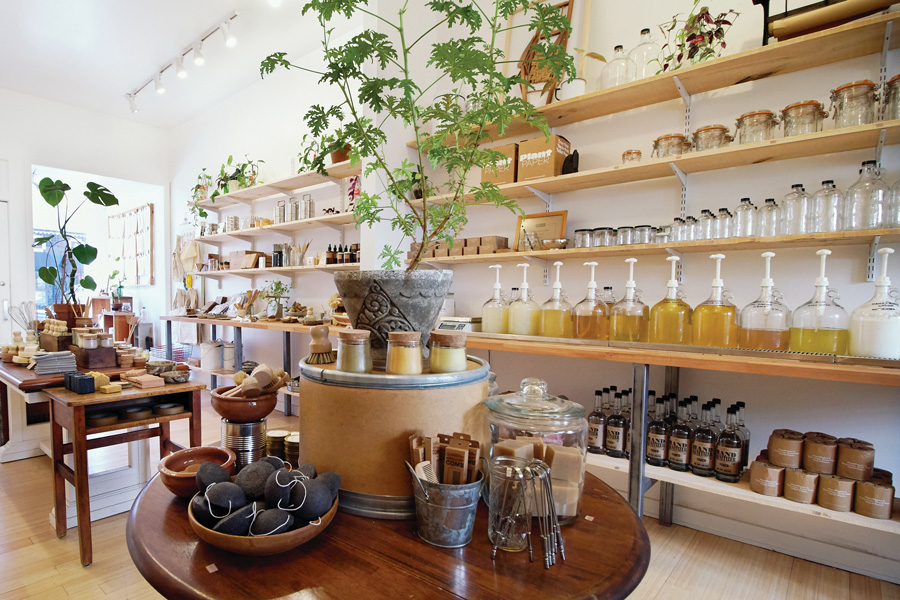The photograph features an apothecary-like shop, bathed in natural daylight and complemented by white overhead lighting. It possesses a warm and inviting ambiance created by an array of wooden shelves that line the walls and display an assortment of wellness and body care items. The shelves are adorned with an eclectic mix of objects, including glass jars filled with mysterious potions, oils, and lotions, and bars of soap. 

In the foreground, a round wooden table is covered with a variety of small items, including decorative elements such as a carved bird and a pedestal holding seasoning bottles. It's flanked by brown paper rolls and full bottles. Several glass jars, resembling cookie jars but filled with soap cubes, enhance the display’s rustic charm. Each table bears a potted plant with green sprouts, adding a touch of nature to the setting.

Dominating the color palette are earthy shades of brown, black, white, gray, green, and accents of yellow and blue. Meanwhile, in the background, a mirror reflects the room’s lively assortment of jars, bottles with pump lids, and additional decorative items, providing a sense of depth and cohesion to the space. The image collectively conveys a serene and well-organized environment, perfect for exploring an array of body and wellness products.